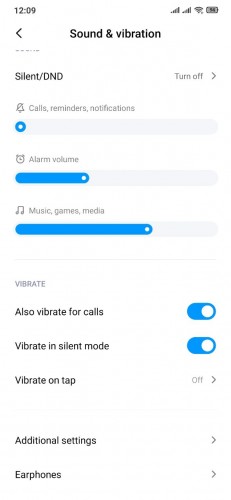This is a mobile screenshot of the "Sound and Vibration" settings menu. The current time displayed in the upper left-hand corner is 12:09. In the upper right-hand corner, icons indicate Wi-Fi strength, cellular signal strength, and battery charge levels.

The header of the settings menu reads "Sound and Vibration," accompanied by a left-facing back arrow on the left side of the text. Below the header, the first option is "Silent / DND" with a right-facing arrow indicating further settings. Currently, the phone's settings allow calls, reminders, and notifications, and this is represented by a volume meter next to a bell icon that is crossed out, indicating that the volume is set to mute. A slider shows that the volume is completely turned down.

Next, the "Alarm Volume," indicated by an alarm clock icon, is set to about one-third of the maximum volume. The "Music, Games, and Media" volume, represented by a music note icon, is set to approximately two-thirds of the maximum volume.

The section labeled "Vibrate" shows that the toggle for "Also vibrate for calls" is turned on, indicated by a blue toggle. Similarly, "Vibrate in Silent Mode" is also activated, showing a blue toggle. The option "Vibrate on tap" is shown to be off.

Overall, this menu allows the user to control various sound and vibration settings, offering a customizable experience for managing different types of audio and vibration alerts.